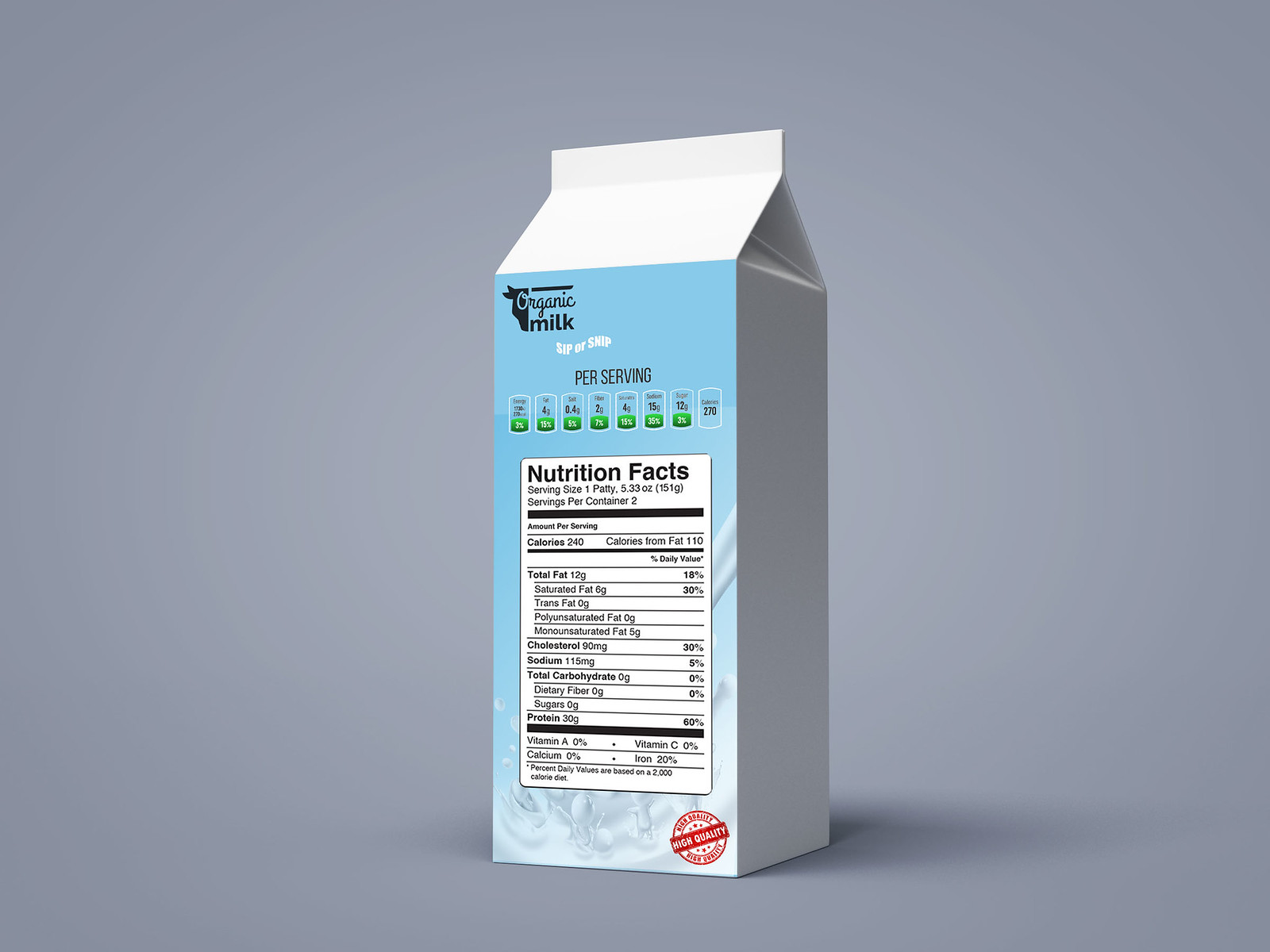This photograph, which appears to be a highly realistic digital 3D rendering, showcases a carton of organic milk set against an indistinct gray background, where the wall and table seem to blend seamlessly. The carton is predominantly light blue with a white top, folded to a point, and features clear branding for organic milk. Prominently displayed is a detailed nutrition facts box, listing 240 calories, 12 grams of fat, 30 grams of protein, and zero carbs, fiber, and sugar per serving. The bottom right corner of the carton is marked with a red quality seal, certifying its high standards. Various badges and logos reinforce its organic authenticity. The carton is angled slightly to the left, and casts a subtle shadow against the background, adding to the realism of the image.